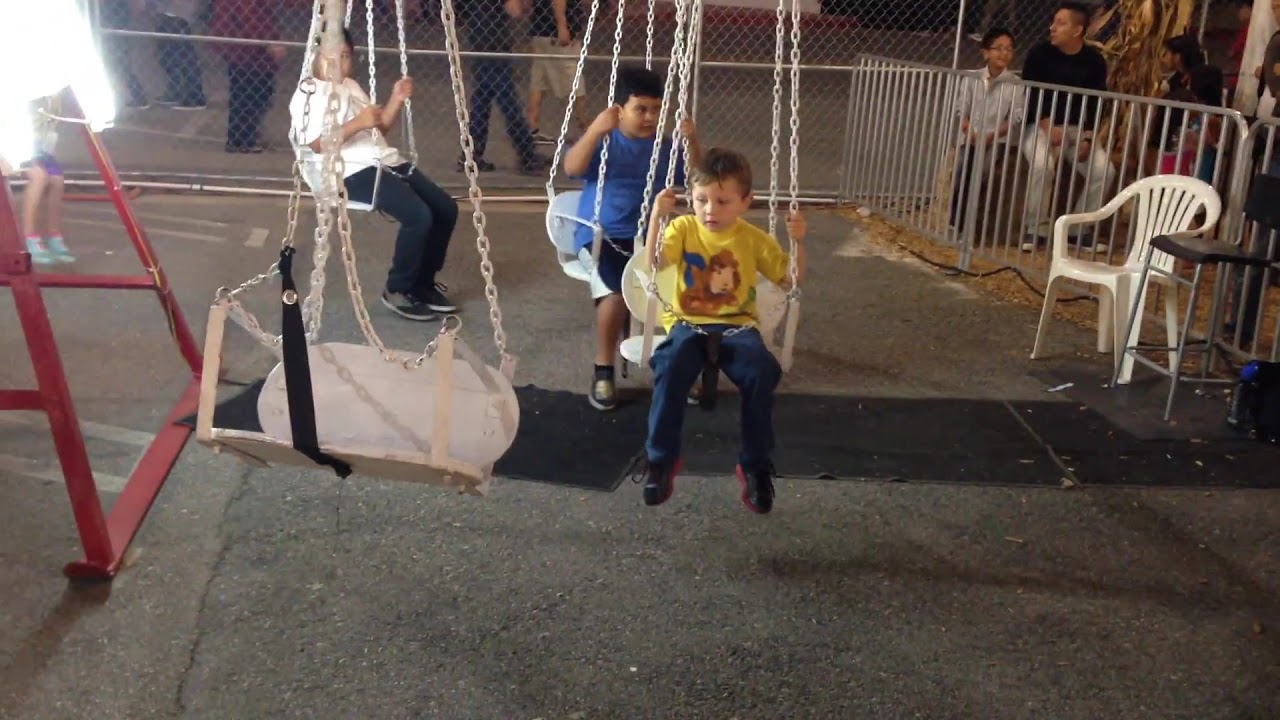In this nighttime photo, we see four children on an amusement ride that appears to be located in a makeshift park or a closed-off parking lot, resembling a county fair or city carnival. The ride features swings suspended by chains, slowly spinning around at about two feet off the ground, enclosed by a fence roughly three and a half feet tall. The first swing on the left is empty, followed by a little boy around five years old with Caucasian skin, wearing a yellow short-sleeved shirt with a guinea pig character on it and dark jeans. Behind him is another boy, around the same age, with light brown skin, sporting a blue t-shirt and black shorts. Further back, a taller boy in a white t-shirt and black pants can be seen coming around the bend. The background reveals a bustling scene with people walking along a main thoroughfare behind a chain-link fence and metal partitions, suggesting a communal, lively atmosphere. Some adults are seated on benches to the right, likely watching their children enjoying the festivities. The area is brightly illuminated by a conspicuous light source in the upper left corner, highlighting the vibrant evening event.